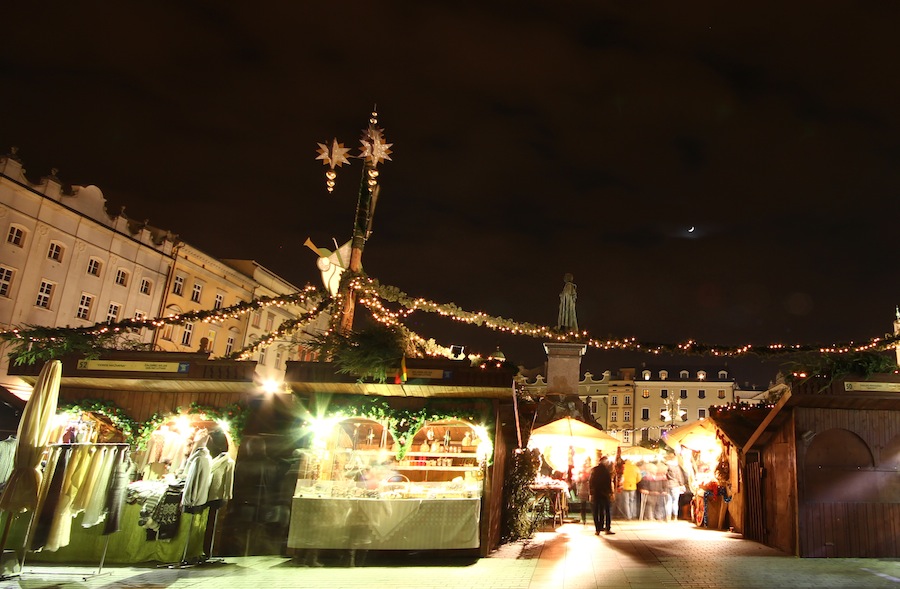This realistic nighttime photograph captures an outdoor Christmas market set in a European town square, framed by 18th to 19th-century style buildings. Under a starless, black sky with a small crescent moon, the market is illuminated by a central pole adorned with strings of green garland wrapped in lights, radiating out to various stalls. These kiosks, some with roofs decorated with green boughs and wreaths, offer an array of items, including clothing and personal care products displayed on hangers and shelves. In the foreground, we see a well-lit stall selling light clothing and what seem to be teas or body products. In the middle area, tables with umbrellas suggest a serving area for drinks, where people are gathered, adding to the festive atmosphere. Prominent in the background, a large statue possibly depicting a Christian leader or Roman figure stands atop a fountain, contributing to the historic ambiance of this bustling holiday market.